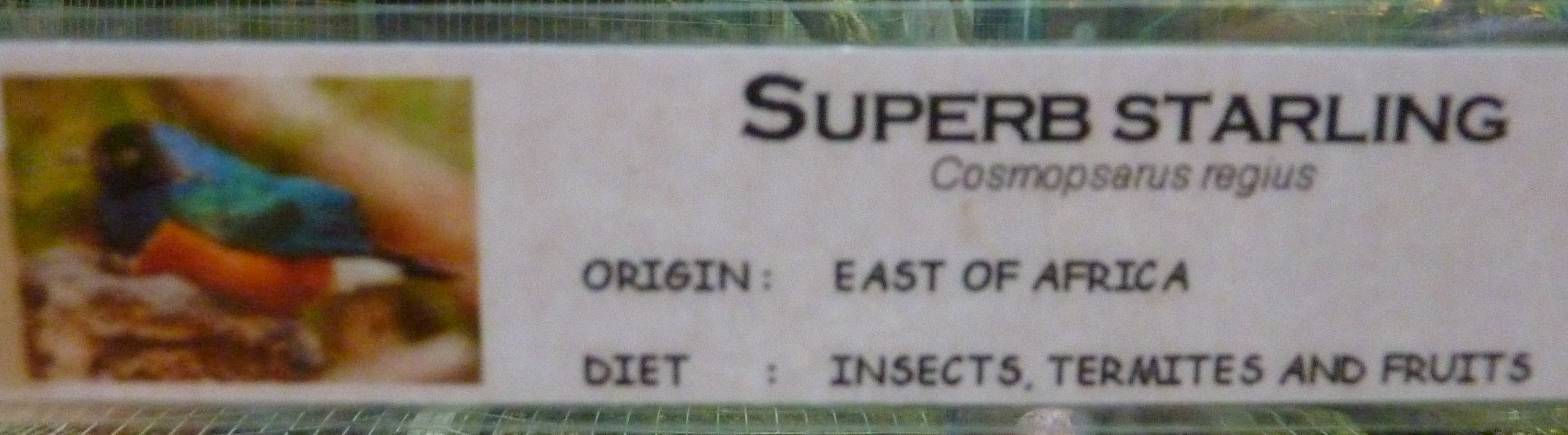The image depicts a laminated sign, likely posted on the side of a cage or enclosure, either in a zoo or a pet store. The sign is a wide, landscape-oriented white rectangle, resembling a sideways bookmark. On the left side of the sign, there is a slightly dark and blurry photograph of a bird, characterized by its blue-green wings, blue breast, dark head, orange underbelly, and a tuft of white and black at the tail end. The bird is perched on a piece of wood or rock, with a tree branch and green leaves of a fern visible in the background. On the right side of the sign, black text identifies the bird as a "Superb Starling," with its scientific name "Cosmosaurus regius" below in italicized gray text. Further information on the sign indicates the starling’s origin as "East of Africa," and its diet comprising "insects, termites, and fruits," marking it as an omnivore.